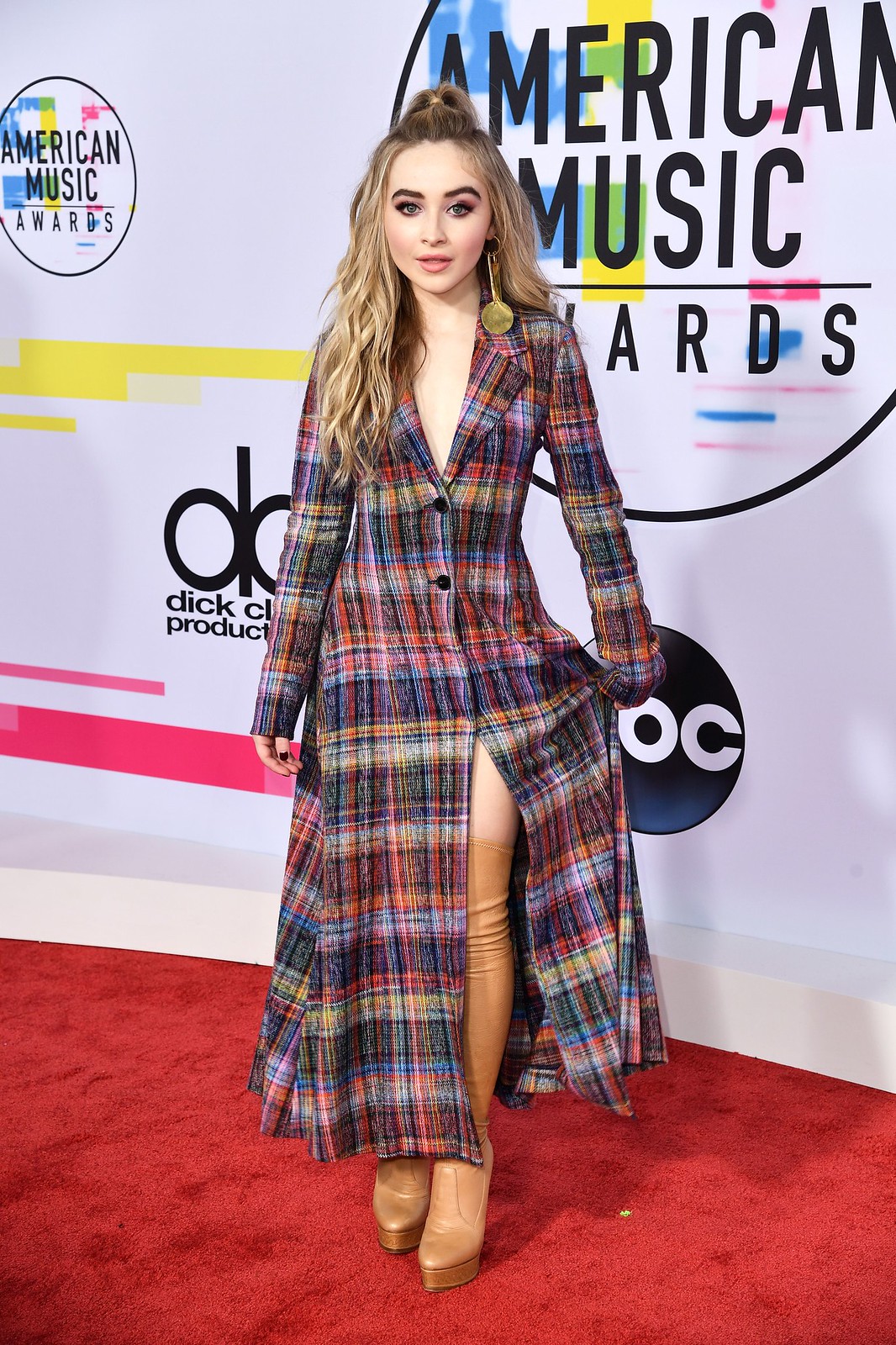In this photograph taken at the American Music Awards, Sabrina Carpenter stands poised on a red carpet, framed against a white backdrop adorned with colorful circular logos and the ABC emblem. Sabrina's outfit is eye-catching: she is draped in a vibrant, plaid trench coat featuring a mix of reds, blues, and yellows. The trench coat is pulled to the side to reveal high-heeled, thigh-high boots in a light brown hue. Her long blonde hair is styled into a ponytail, with free-flowing strands cascading over her shoulders, particularly on the left side. She accessorizes with large gold dangle earrings and subtle eyeshadow that accentuates her features. Sabrina gazes directly ahead, effortlessly commanding attention as she poses for the paparazzi amidst the lively atmosphere of the event.